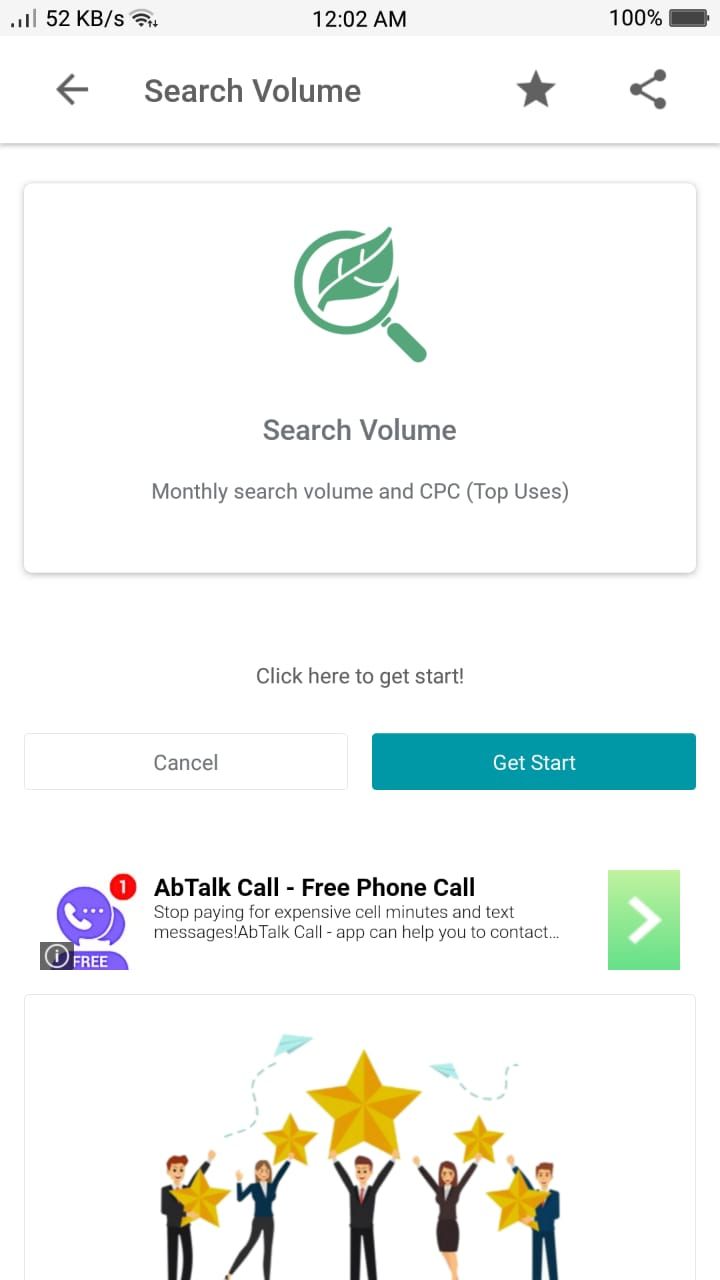The image captures the interface of a website, featuring a user-friendly and visually structured design. 

At the very top, there is a light gray banner displaying various status indicators: on the left, a cell signal symbol next to "52KB/s", a Wi-Fi signal icon, and a pair of small up-and-down arrows. Centrally positioned on the banner is the current time displayed as "12:00 AM". On the right side, a battery icon shows a full charge at "100%".

Below the banner, the main content area has a clean white background. On the left side, there is a leftward arrow, presumably for navigation. Next to it, the interface includes a search volume graphic, a star icon, and a share button. Beneath these, there is a rectangular section with a distinctive green magnifying glass icon, embellished with a leaf, indicating an environmentally-friendly search volume feature. Text within this section reads "Search Volume" with additional metrics like CPC displayed in parentheses, labeled as "top uses."

Further down, a prominent call-to-action button urges users to "Click Here to Get Started!" This section is flanked by two smaller buttons: "Cancel" on the left, and the teal-blue "Get Start" button on the right.

Continuing downward, the site introduces "AB Talk Call - Free Phone Call." Accompanying this section is a purple circular icon, illustrated with a telephone symbol and marked with a red notification badge displaying the number "1". This feature is highlighted as being free. 

Adjacent to this, there's a green leftward arrow next to a cream-colored square containing a white rightward triangle. Underneath, five illustrations of people holding gold stars convey user approval or ratings. 

Overall, the website interface is detailed, intuitive, and adorned with various interactive elements designed to engage users effectively.